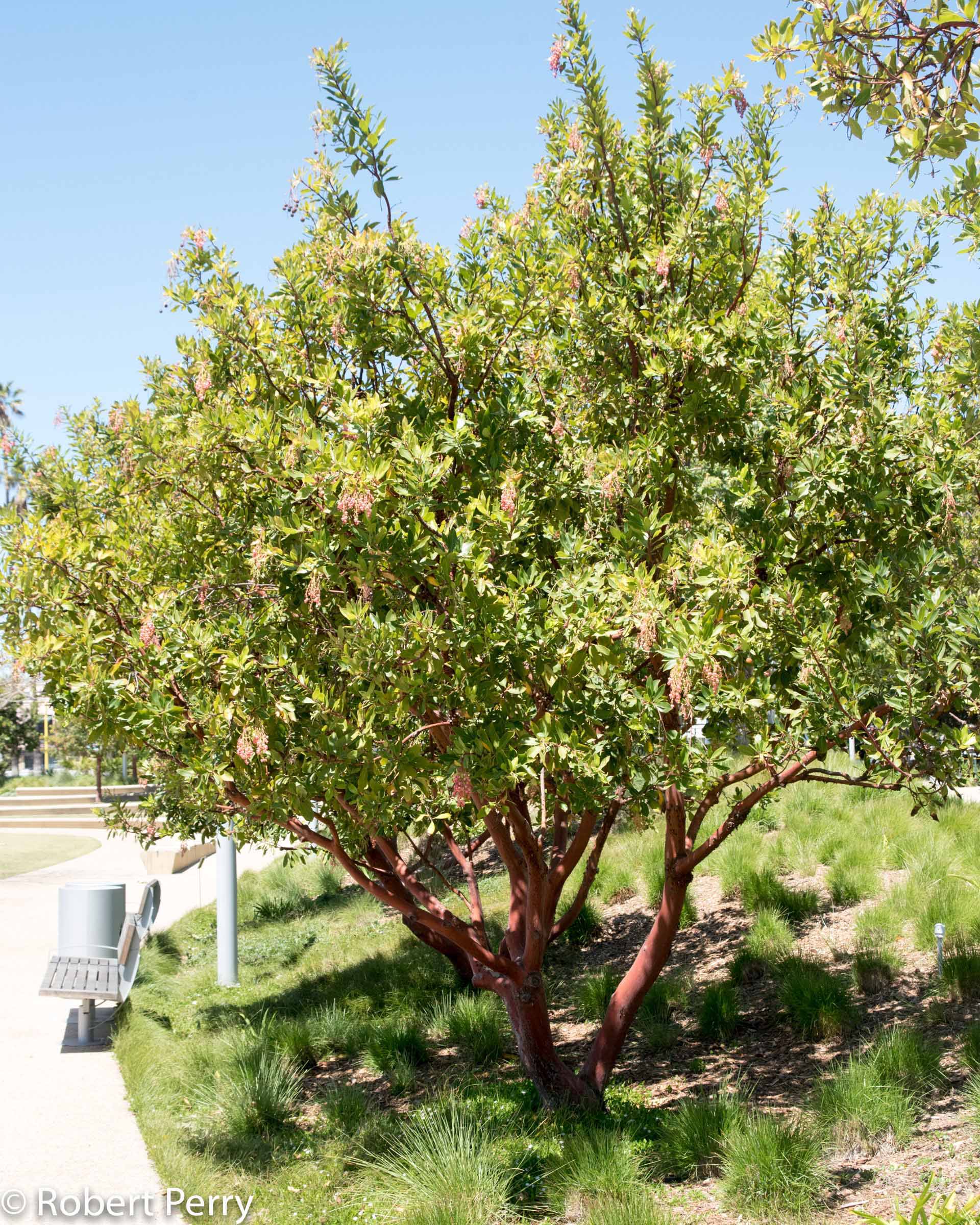This color photograph captured by Robert Perry features a large, blooming tree with abundant green leaves and eye-catching sprays of reddish flowers. The tree's slender trunk and branches are a striking deep reddish-brown, suggesting it might be a manzanita tree. The base of the tree is surrounded by clumps of lush green grass. Behind the tree, a clear blue sky stretches without a cloud in sight, providing a tranquil backdrop. To the left of the tree, within a park setting, a wooden bench and a metal trash can are situated near a sidewalk. The photograph also includes a noticeable path running from the forefront to the rear of the image, bordered by a series of steps in the background. A copyright notice in white, indicating "Robert Perry," is present in the bottom left corner, attributing the photograph to him.